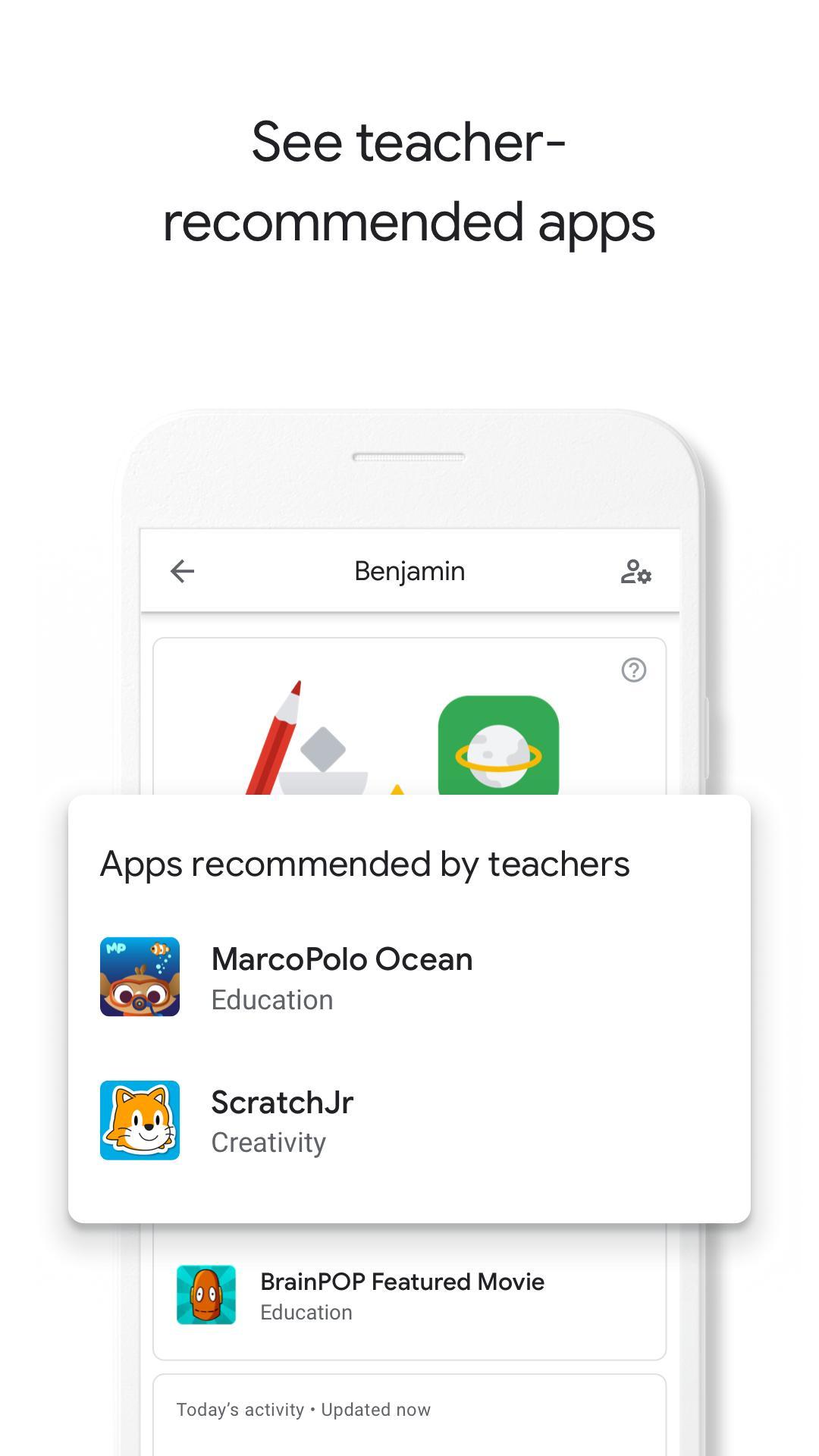In the image, the top section features the text, "See Teacher Recommended Apps." Below this, there is a light blue smartphone displayed against a white background, intersected by a white line. On the screen of the smartphone, there is a left-facing arrow next to the name "Benjamin," accompanied by small icons representing people. 

Further down the screen, there are several elements: a red pencil lying next to a couple of small gray blocks, a green box featuring a white globe with a yellow ring around it, and an additional box displayed prominently in the foreground with the text "Apps Recommended by Teachers."

The highlighted apps included are "Marco Polo Ocean," categorized under educational apps, and "Scratch Junior," aimed at fostering creativity. Icons or thumbnails for these apps are also displayed in small boxes. Another featured item is “Brain Pop Featured Movie,” indicated by its own thumbnail image. 

At the bottom, two blue horizontal lines demarcate a separate section, which notes "Today's Activity Updated Now." This section reinforces the availability of teacher-recommended apps, prominently featuring Marco Polo Ocean for education, Scratch Junior for creativity, and Brain Pop as a featured movie for further learning and engagement.